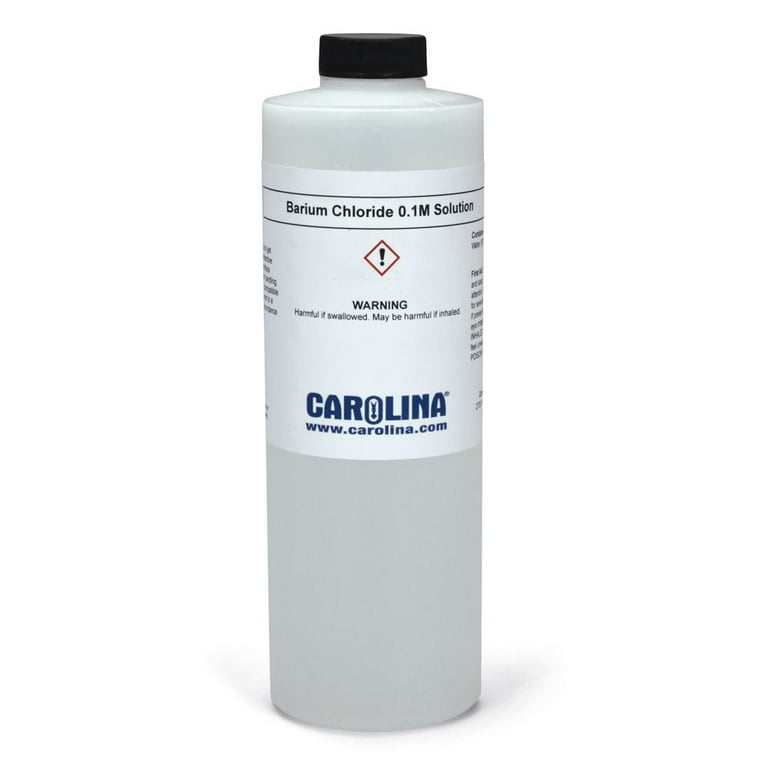This photograph features a tall, cylindrical white bottle standing upright against a plain white background, creating the illusion of the bottle floating in mid-air. The bottle has a clean, modern white label that is a clearer, brighter white than the bottle itself. At the top of the bottle, there is a black screw-on lid. The label prominently displays in black text "Barium Chloride 0.01M solution." Directly below this text is a red diamond shape with a black exclamation point, followed by a warning in black font that reads: "WARNING: Harmful if swallowed. May be harmful if inhaled." Lower on the label, the name "Carolina" and the website "www.carolina.com" are printed in blue text. Small, cut-off black text is visible on the left and right sides of the label. The overall composition is minimalistic, with no additional imagery, people, or colors other than the black, red, and blue text and iconography mentioned. A slight shadow behind the bottle provides a subtle depth to the image.